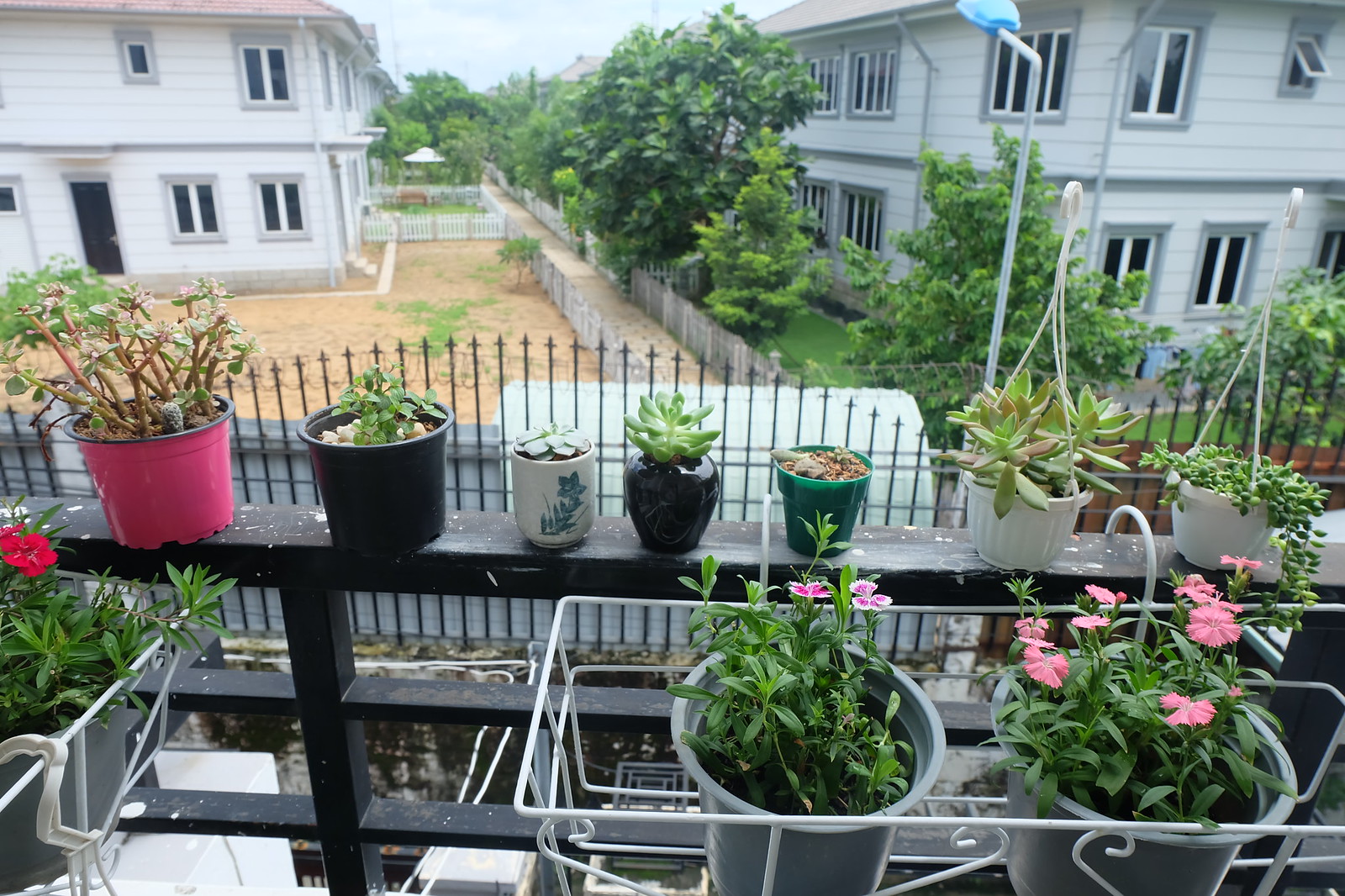The photograph features a close-up view of a variety of potted plants arranged on a tall, black balcony railing, with additional plants resting on white wire frames. The balcony belongs to an outdoor patio area, showing some spots of white paint or chipped wood. The plants show a diverse assortment, including colorful flowers and cacti. Notably, there are:

1. A black pot with green leaves and blooming red flowers.
2. A gray pot containing green leaves and pink flowers with violet centers.
3. Another gray pot filled with green leaves and blossoming pink flowers.

In the background, the photograph captures two neighboring homes separated by wooden fences. The house on the viewer's left is primarily white and has a yard with patches of brown grass, reflecting a more barren landscape with some green spots and possibly a bush. In contrast, the house on the right is primarily gray, boasting lush green grass and several flourishing trees. The overall ambiance evokes a peaceful outdoor patio area with a striking contrast between the two adjacent yards.